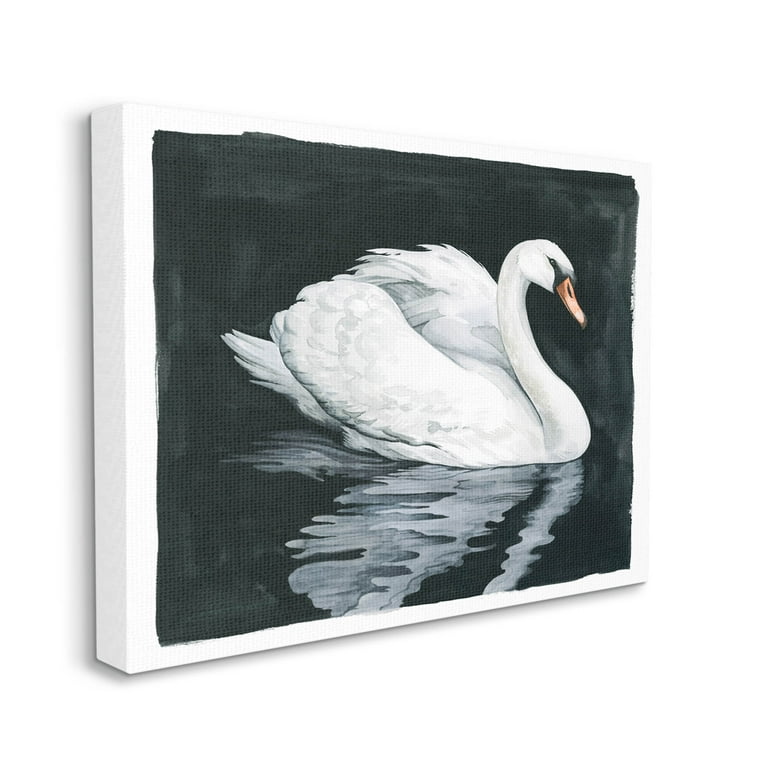A canvas painting depicts a serene scene of a white swan floating gracefully in a textured, near-black pond. The swan, characterized by its white plumage and yellow-orange beak, faces right with its head slightly down and its wings tucked neatly behind. A subtle reflection of the swan can be seen in the rippled water, adding depth to the composition. The painting is bordered by a roughly half-inch white margin around the edges of the canvas, contrasting with the dark background. The jagged edges of the black background add an abstract touch, hinting at a night setting. The canvas itself hangs on a white wall with a dark drop shadow accentuating its presence.